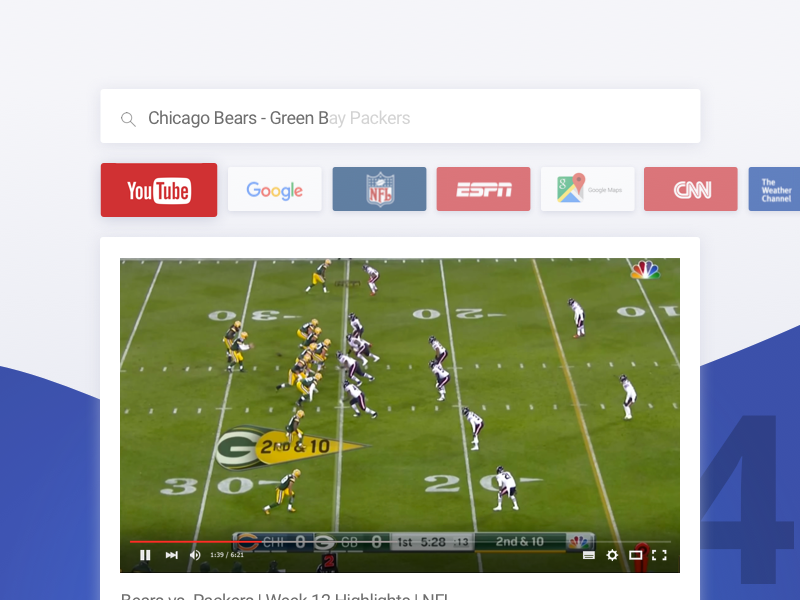In a vibrant, visually engaging image resembling a digital football field, the background is predominantly green, symbolizing the turf. In the foreground, the bottom corners are tinted blue. Prominently displayed are four lines of logos and text: "Chicago Bears," "Green Bay Packers," "Red Fang," "Osceola," "Square Enix," "YouTube," "Google," "NFL," "Google Squared," "ESPN," "Google Maps," "CNN," "The Weather Channel," indicating various entities likely associated with a sporting event or broadcast. At the very top right, the iconic NBC Peacock logo is visible, suggesting network affiliation.

The center of the image features a video player interface with the controls clearly labeled: 'Pause' on the bottom left, a speaker icon revealing '139 out of 621,' a 'Caption' option, a 'Gear' symbol for settings, and a 'Square' possibly for full-screen mode. The video player hints at football content, further supported by field markings reading "30, 20, 10," alongside text indicating "second and 10," enhancing the sports theme. The overall array of logos, symbols, and text elements align to create a comprehensive, lively representation of a football-related broadcast or digital interface.